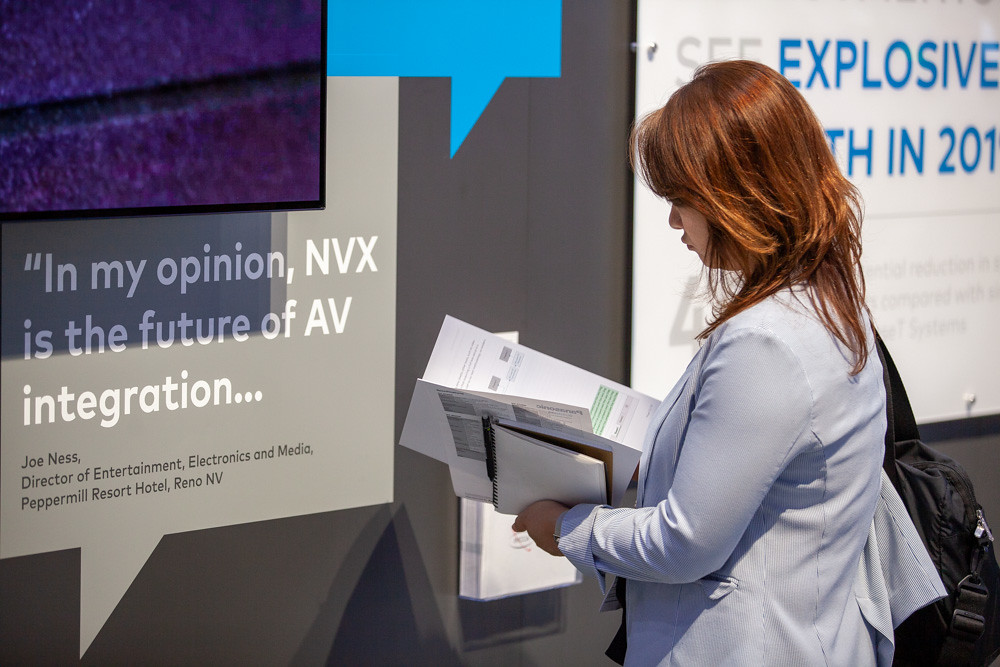A woman with reddish-brown hair, wearing a light blue long-sleeve shirt with the cuffs rolled up, is seen intensely focused on reading several envelopes and papers she's holding. Her face is obscured by her hair and the angle of the photograph. She's standing in a setting where a black backpack hangs over her right shoulder. Behind her, there's a sign that reads "In my opinion, NVX is the future of AV integration," attributed to Joe Ness, Director of Entertainment, Electronics, and Media at Peppermill Resort Hotel in Reno, Nevada. The sign appears to be in a square dialogue box format. The woman seems deeply engaged with the mail she's examining.